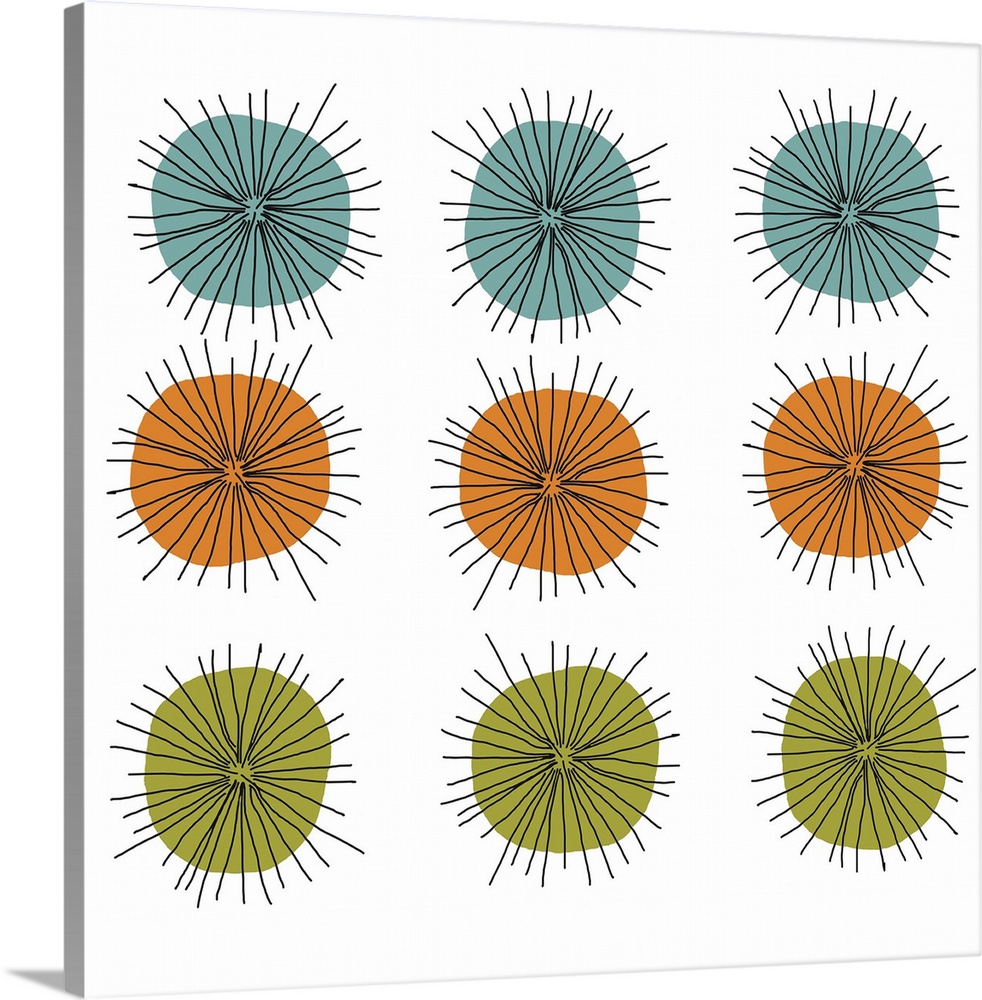This digital image shows a white canvas featuring a meticulously arranged grid of nine painted objects, organized in three rows and three columns. The objects, which resemble circular forms with irregular edges, occupy a backdrop that appears grey due to the shading effects on the left and bottom left of the image. The top row is adorned with three turquoise circles, each displaying black hair-like lines radiating from their center in a sunburst pattern. The middle row contains three orange circles with a similar design, and the bottom row features three olive green circles. Each painted object is unique, as the sunburst patterns slightly differ, adding variation amidst the consistent grid layout. The overall aesthetic suggests a stock image or a decorative print often found in home goods stores, with a digital rendering evident from the distinctly artificial shadowing.